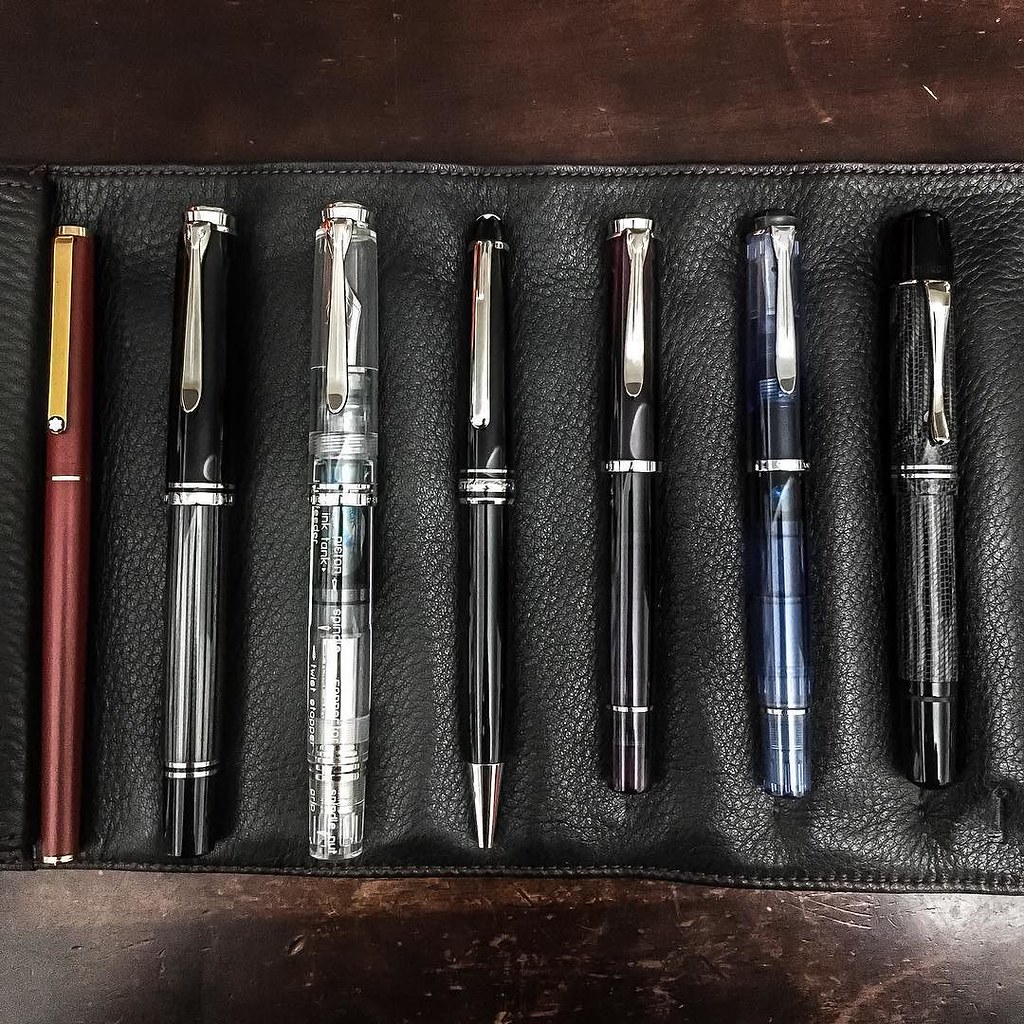This horizontal rectangular photograph showcases a refined collection of seven intricately designed writing pens, artfully laid out on a black leather pouch with visible stitching at the top and bottom, unrolled atop a dark brown, wood-grain table. Each pen, suggesting an air of sophistication and expense, is meticulously arranged from left to right. The first pen is a striking burgundy with a gold clip, exuding a classic elegance. Next is a pen featuring a sleek black top, a silver body, and a black end. Following is a transparent pen displaying the inner mechanisms and labeled "ink tank spindle," set off with black and silver accents. Adjacent is a slim black pen with silver clips and a polished point, radiating simplicity. Beside it, a slightly shorter black pen with no visible tip and adorned with a silver handle. Included is a pen with a dynamic blue body, accented by a distinctive black and white stripe and finished with a silver hook. Concluding the range is a robust black pen with subtle gray elements and a silver pocket clip, rounding off this elegant assembly.